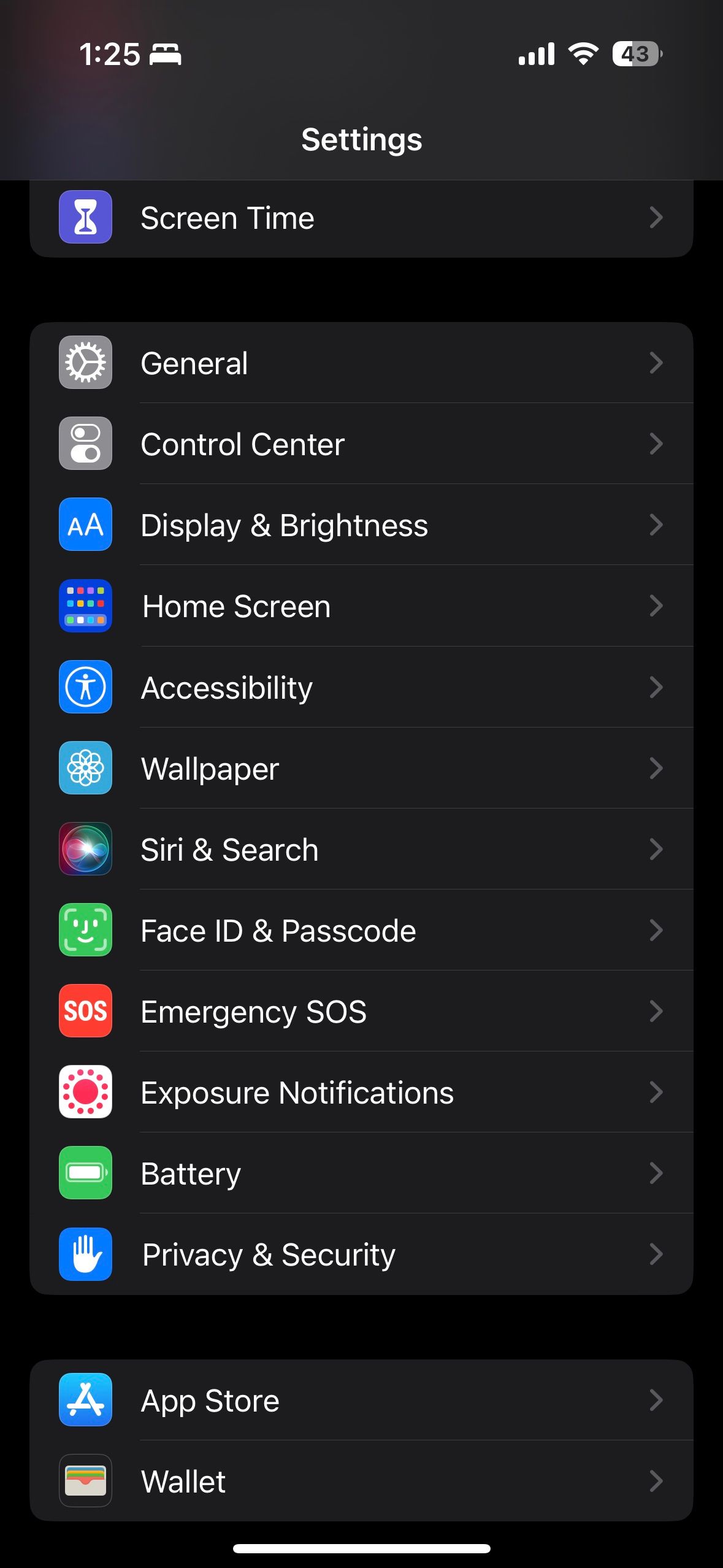The image is a screenshot from an iPhone, displaying the Settings app interface. At the top left corner, the time is shown as 1:25, accompanied by a small bed symbol. The status bar indicates full cellular service with four bars, a strong Wi-Fi connection with three full bars, and the battery level is at 43%. The Settings menu is laid out with several options listed:

- At the top, "Screen Time" is visibly separated from the other sections.
- The next section includes: "General," "Control Center," "Display & Brightness," "Home Screen," "Accessibility," "Wallpaper," "Siri & Search," "Face ID & Passcode," "Emergency SOS," "Exposure Notifications," "Battery," and "Privacy & Security."
- Following another break, the final section lists "App Store" and "Wallet."

Each setting has a corresponding gray arrow on the right-hand side, indicating that selecting it will open additional information or options. On the left-hand side, each setting is paired with a corresponding icon that visually represents the setting title.